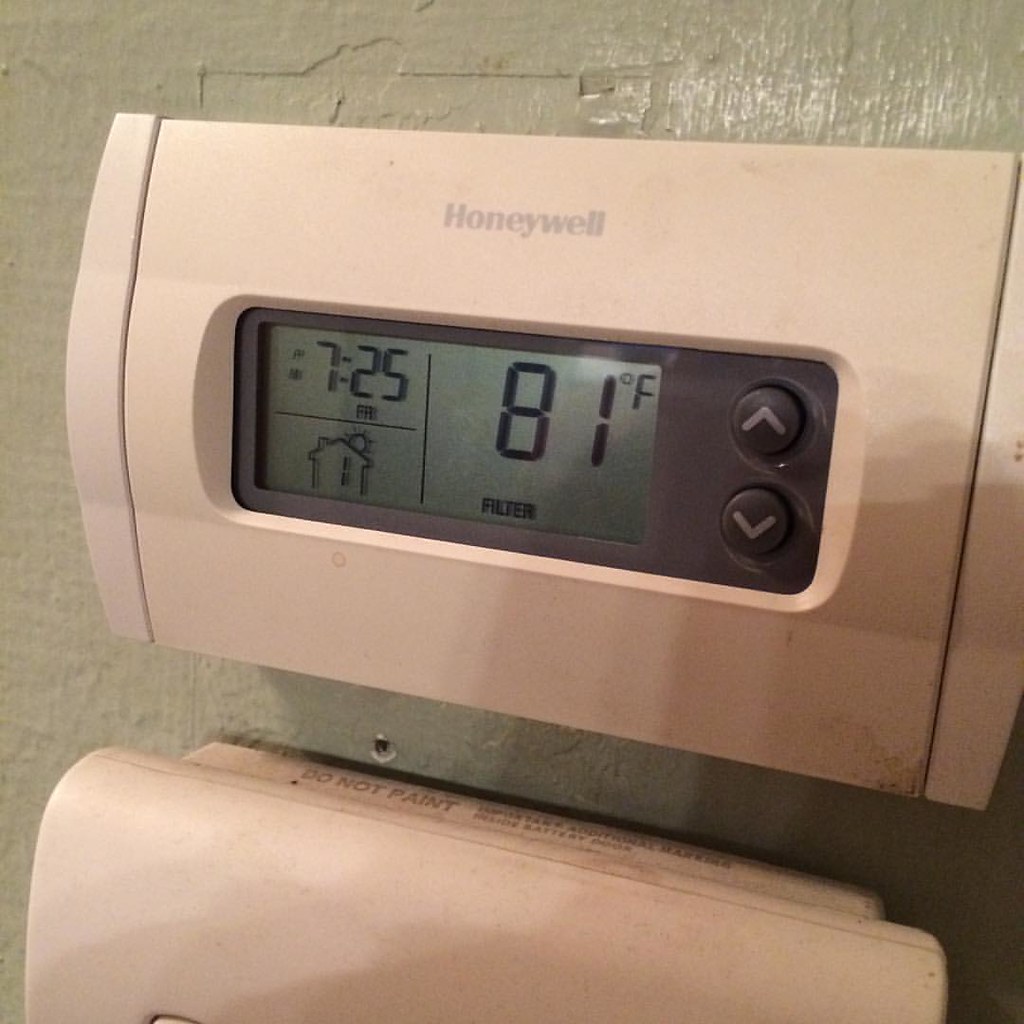A light brown concrete wall serves as the backdrop for a prominently displayed Honeywell thermostat. This thermostat is light pink in color and features gray writing. An oblong window on the thermostat showcases the time, "7:25 AM," alongside an icon of a house with a dotted line to its right. Below this window, the current temperature is displayed as "81°F," accompanied by the word "filter." The thermostat also includes black up and down buttons with pink print to adjust the settings. About an inch beneath the thermostat, there's a small nail hole. Beneath this, another pink box of a similar size is mounted on the wall. However, its function remains unclear—it could be another thermostat or a different kind of control device.